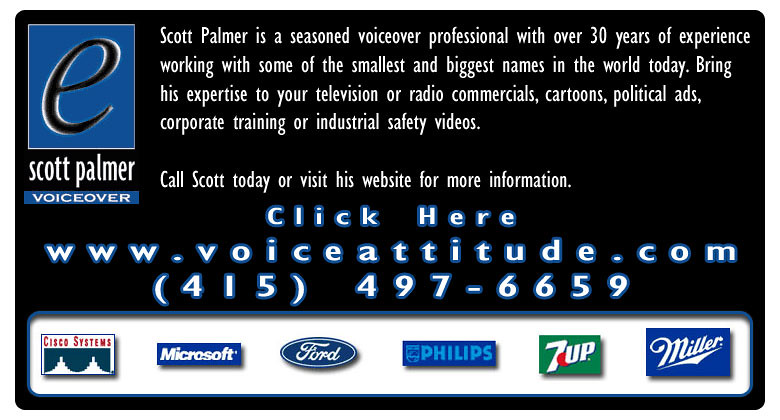The image displays an advertisement for voice-over artist Scott Palmer. On the left side, there is a prominent letter "E" on a blue background with "Scott Palmer Voiceover" written beneath it. The top of the image features white text on a black background, introducing Scott Palmer as a seasoned voice-over professional with over 30 years of experience. It highlights his expertise in working with a diverse range of clients, from independent ventures to globally recognized corporations. The text encourages potential clients to leverage his skills for television or radio commercials, cartoons, political ads, corporate training, and industrial safety videos. It invites viewers to contact him through his website, www.voiceattitude.com, or by phone at 415-497-6659. The bottom of the image showcases icons of notable companies Scott Palmer has collaborated with, including Cisco Systems, Microsoft, Ford, Philips, 7-Up, and Miller, underscoring his extensive professional background.